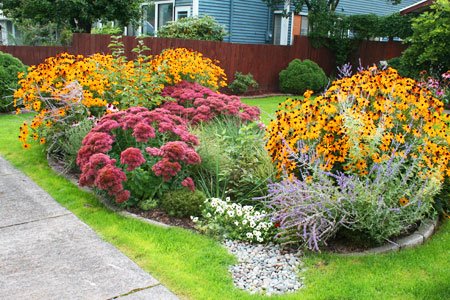This photo showcases a beautifully maintained front lawn garden set in a suburban neighborhood. The garden is prominently outlined by gray-brick-like stones, forming a roughly oval-shaped flowerbed amidst a lush, green lawn. In the foreground, striking black-eyed Susans with their bright yellow petals and dark centers dominate both ends of the garden. Complementing them are patches of fragrant lavender and clusters of smaller white flowers that resemble daisies. Adding to the vibrant display are larger pink flowers, possibly of a rosy variety, contributing to the rich palette of the garden. 

Towards the background, there is a brown wooden fence lined with bushes along the property line, creating a sense of privacy. Behind the fence stands a blue, wooden-clad house partially obscured by the branches of a tree. The detailed layering of plants and thoughtful design of the space indicates a well-tended garden that likely belongs to a home in a coastal region, possibly in northeastern America.